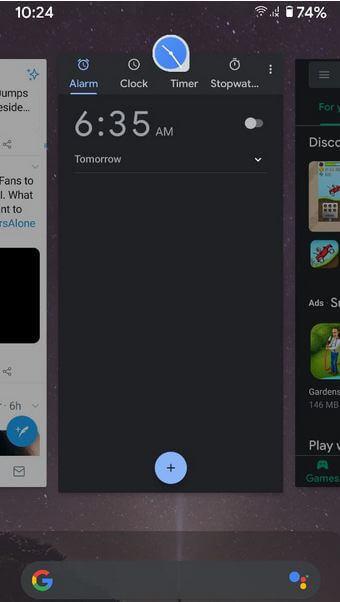The screenshot displays an Android device with the open apps interface visible. At the bottom, there's a Google search bar featuring the recognizable "G" logo on the left and four colored dots (blue, red, yellow, and green) on the right. The search bar itself is currently empty. 

In the center of the screen, the alarm clock app is open, showcasing a detailed interface. At the top, a clock icon indicates the current time as 10:20. The alarm section displays a digital format of 6:35 AM set for the next day, which is currently toggled off. Below, options for Clock, Timer, and Stopwatch are visible but not in use. The primary view is set against a dark background, emphasizing the minimalist design.

To the left, there's a partially visible news app, suggesting the user can scroll horizontally to access different apps. To the right, an undetermined game-related app or game store is open but not fully recognizable. This interface rests on a wallpaper that depicts a night sky, speckled with what seems to be stars and possibly a faint light from the ground, adding a whimsical touch to the view.

The clock at the top of the screen is encased in a white circle, converging into a teardrop shape on its lower right-hand side, creating a distinctive design feature.